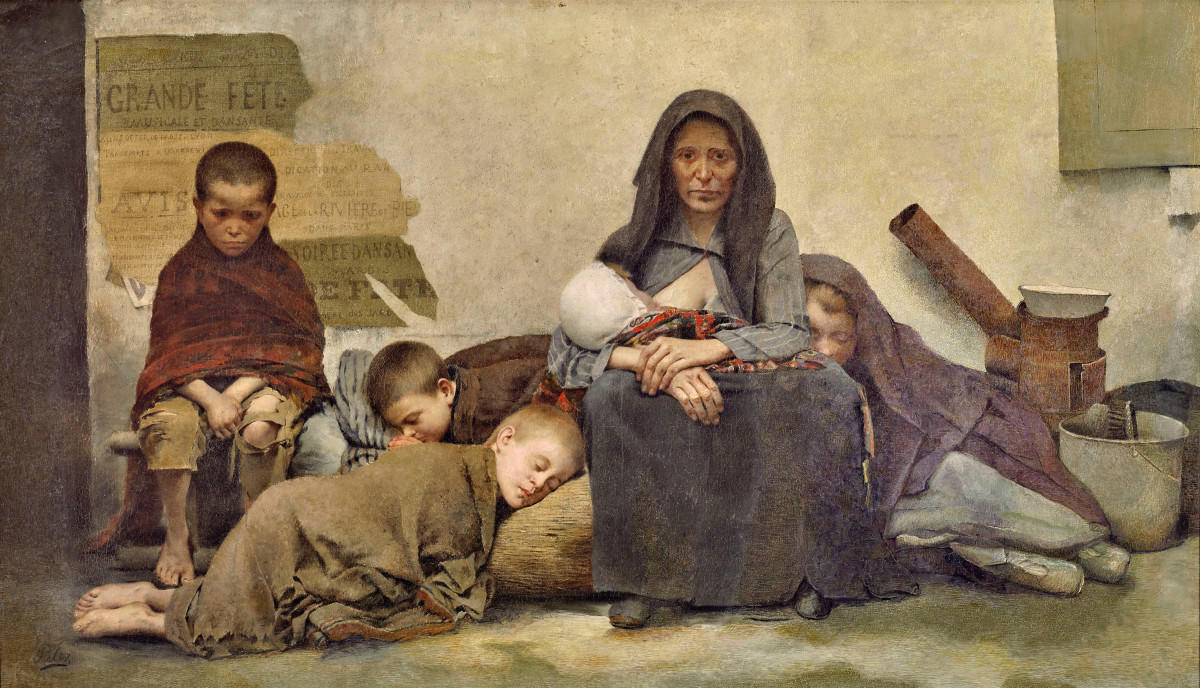This horizontal rectangular painting, titled "Sans Asile" by Fernand Pelez, created around 1880, vividly portrays the poignant scene of a destitute homeless family. The artwork, executed with such realism that it almost resembles a photograph, is rich in color and detail. The central figure is a woman sitting on a grayish-brown sidewalk, leaning against a cream-colored stucco building. She exudes a sense of despair as she gazes beseechingly at the viewer while holding an infant, whom she may be nursing. Her attire includes a dark, scarf-like cloth around her head, a gray shirt that is open for breastfeeding, and a long, dirty purple skirt that reaches the ground.

Surrounding the woman are four children, who appear to be sleeping. On her right, a young girl rests her head on the woman's lap, partially covered by a purple blanket. To her left, in the foreground, lies a young boy on a pillow, wrapped in a brown blanket with his feet extending towards the bottom left corner of the painting. Behind this boy, two other boys are positioned; one is seated with a red blanket draped around his shoulders, while the other lies asleep beside him on a pillow.

The setting is an alley filled with a mixture of debris and personal belongings, symbolizing the harsh reality of their existence. There are items such as a bucket, a piece of wood with a handle, rusted stovepipes, ceramic pots and urns, and dirty dishes scattered around. Attached to the wall behind them are torn and faded signs, possibly old newspapers or posters, adding to the scene's air of decay and neglect. The family members are barefoot, further emphasizing their poverty and hardship. This detailed and sorrowful depiction captures the grim reality faced by many during that era, making it a powerful commentary on homelessness and poverty.